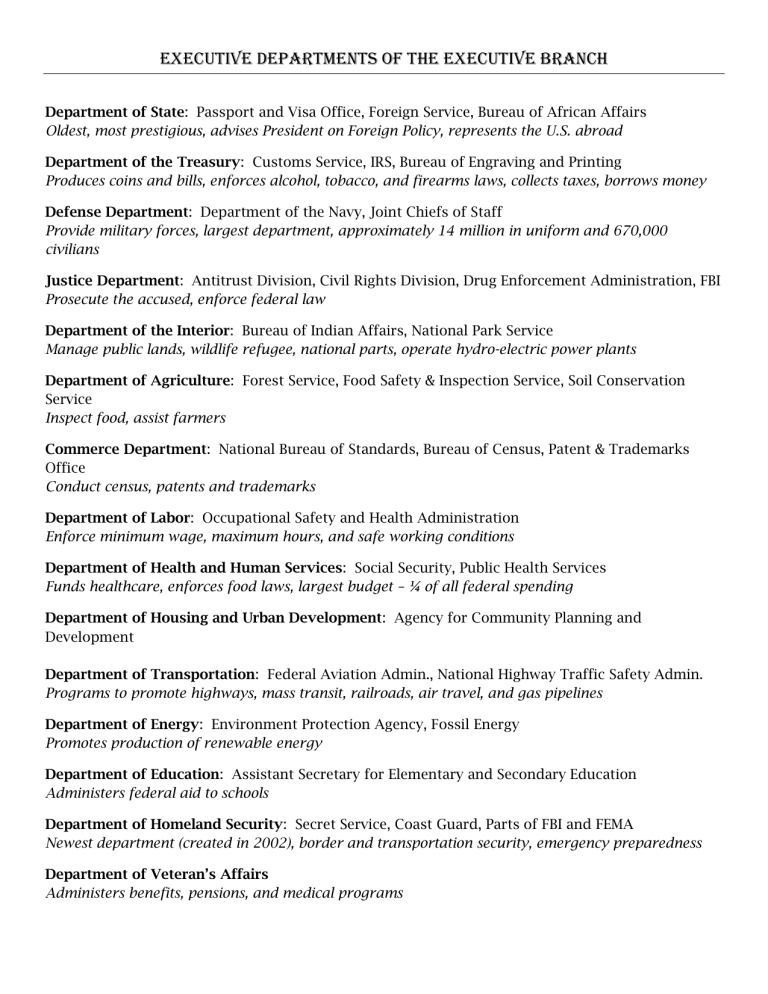The image depicts a white document that provides a comprehensive list of the executive departments under the executive branch of the United States government. Each department name is bolded, followed by an italicized description, while the rest of the text appears in normal print. The document organizes and explains the functions of each department as follows:

- **Department of State**  
  _Passport and Visa Office, Foreign Service, Bureau of African Affairs_  
  The oldest and most prestigious department, it advises the president on foreign policy and represents the United States abroad.

- **Department of the Treasury**  
  _Customs Service, IRS, Bureau of Engraving and Printing_  
  Responsible for producing coins and bills, enforcing alcohol, tobacco, and firearm laws, collecting taxes, and borrowing money.

- **Department of Defense**  
  _Department of the Navy, Joint Chiefs of Staff_  
  Provides military forces and is the largest department with approximately 14 million personnel in uniform and over 670,000 civilians.

- **Department of Justice**  
  _Antitrust Division, Civil Rights Division, Drug Enforcement Administration, FBI_  
  Prosecutes the accused and enforces federal law.

- **Department of the Interior**  
  _Bureau of Indian Affairs, National Park Service_  
  Manages public lands, wildlife refuges, and national parks, and operates hydroelectric power plants.

- **Department of Agriculture**  
  _Forest Service, Food Safety and Inspection Service, Soil Conservation Service_  
  Inspects food and assists farmers.

- **Department of Commerce**  
  _National Bureau of Standards, Bureau of Census, Patent and Trademarks Office_  
  Conducts the census and manages patents and trademarks.

- **Department of Labor**  
  _Occupational Safety and Health Administration_  
  Enforces minimum wage, maximum hours, and safe working conditions.

- **Department of Health and Human Services**  
  _Social Security, Public Health Services_  
  Funds health care, enforces food laws, and maintains the largest budget, accounting for a fourth of all federal spending.

- **Department of Housing and Urban Development**  
  _Agency for Community Planning and Development_ 

- **Department of Transportation**  
  _Federal Aviation Administration, National Highway Traffic Safety Administration_  
  Promotes highways, mass transit, railroads, air travel, and gas pipelines.

- **Department of Energy**  
  _Environment Protection Agency, Fossil Energy_  
  Promotes the production of renewable energy.

- **Department of Education**  
  _Assistant Secretary for Elementary and Secondary Education_  
  Administers federal aid to schools.

- **Department of Homeland Security**  
  _Secret Service, Coast Guard, parts of the FBI and FEMA_  
  The newest department, created in 2002, responsible for border and transportation security, and emergency preparedness.

- **Department of Veterans Affairs**  
  _Administers benefits, pensions, and medical programs to veterans._

This detailed breakdown provides insight into the roles and responsibilities of each executive department.